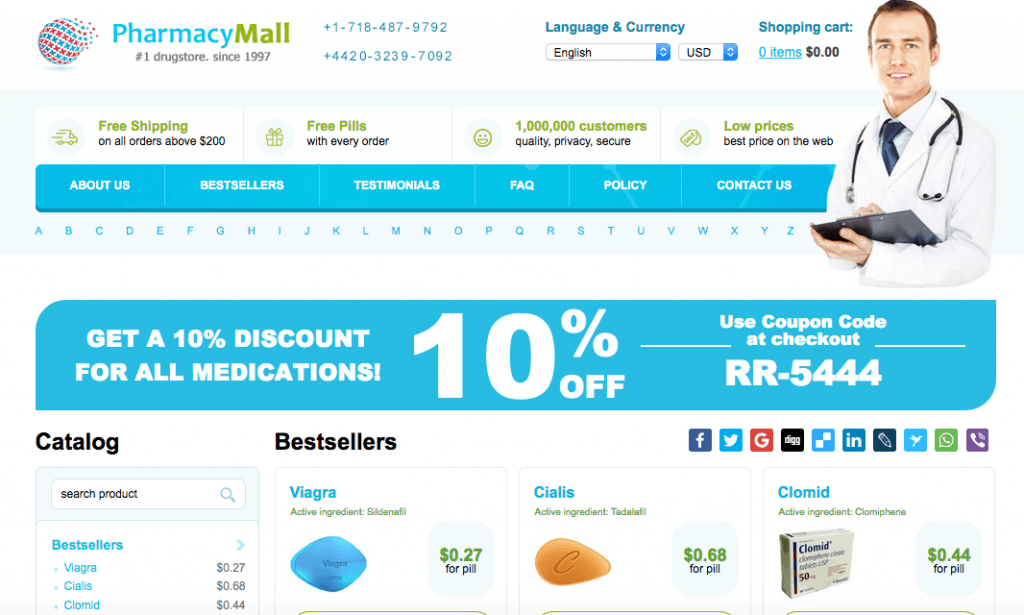"At the top of the image, a banner prominently displays 'Pharmacy Mall, Number One Drugstore Since 1997,' followed by contact numbers: +1-718-487-9792 and +44-203-239-7092. The language is set to English, and currency is USD. The shopping cart icon shows '0 items, $0,' accompanied by a promotional message: 'Free Shipping on All Orders Over $200' and 'Free Pills with Every Order.' Below this, it highlights a customer base of 'a million customers' and reassures with statements like 'Free Privacy,' 'Secure,' 'Low Prices,' and 'Best Price on the Web.'

Directly underneath, a navigation menu includes links: 'About Us,' 'Best Sellers,' 'Testimonials,' 'FAQ,' 'Policy,' and 'Contact Us.' This section is followed by an alphabetical index (A-Z). Additionally, there's a promotional offer: 'Get a 10% Discount on All Medication' with the code 'RR-5444' to be used at checkout. At the bottom, social media icons for Facebook, Twitter, Google+, and LinkedIn are displayed."